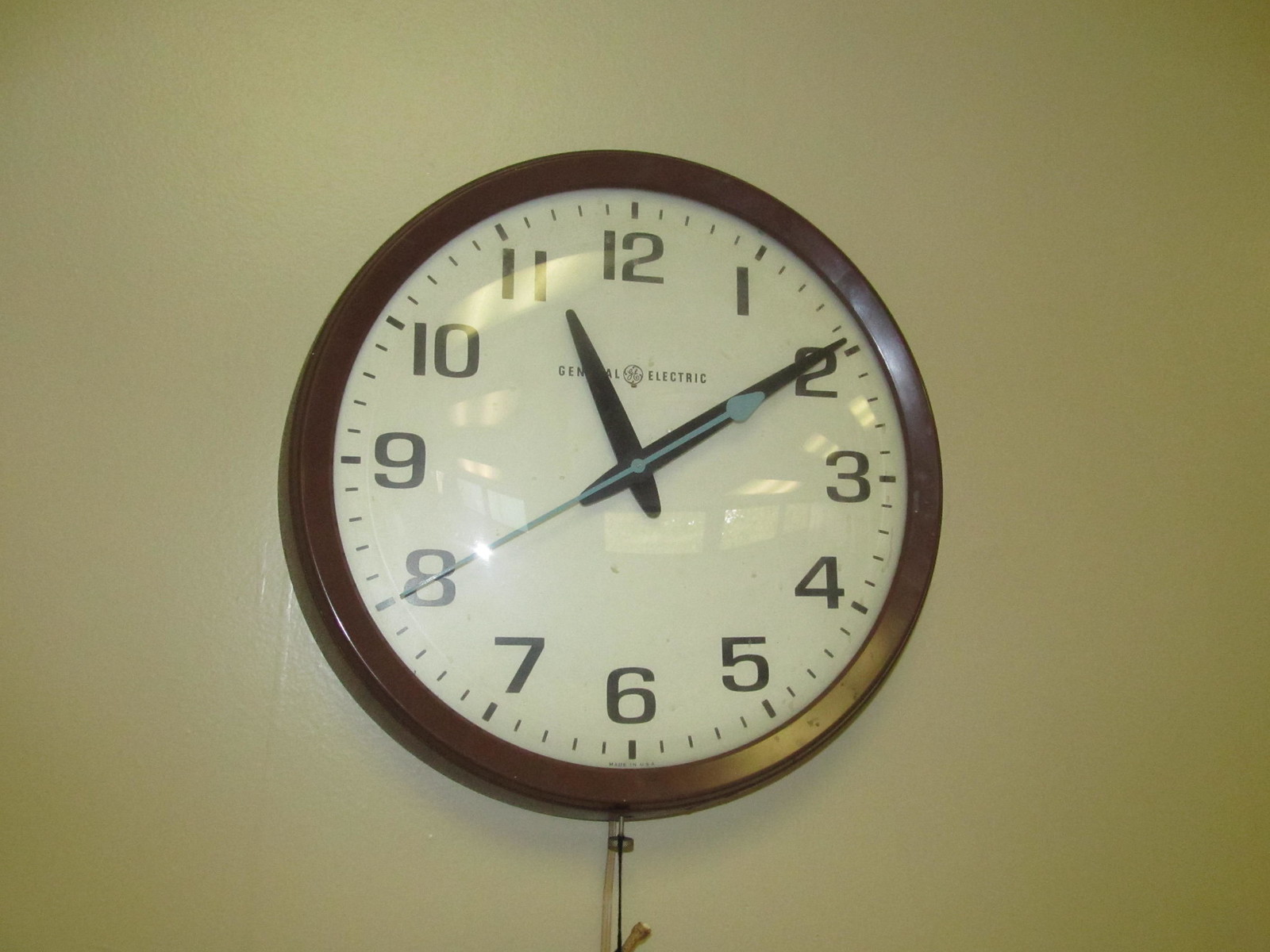The image depicts a circular wall clock hanging on what appears to be a white wall. The clock has a dark brown, reflective border that seems to be made of either plastic or metal. The face of the clock is white with black numbers ranging from 1 to 12, accompanied by minute markers. The hour and minute hands are black, while the second hand is a light blue color. The time displayed on the clock is 11:09 and 40 seconds. The brand "General Electric" is prominently featured in the center, with a logo displaying the letters "GE" in script within a circle. There is a faint reflection on the clock, suggesting windows or an outside view. At the bottom of the clock, there appears to be an indistinct object hanging.